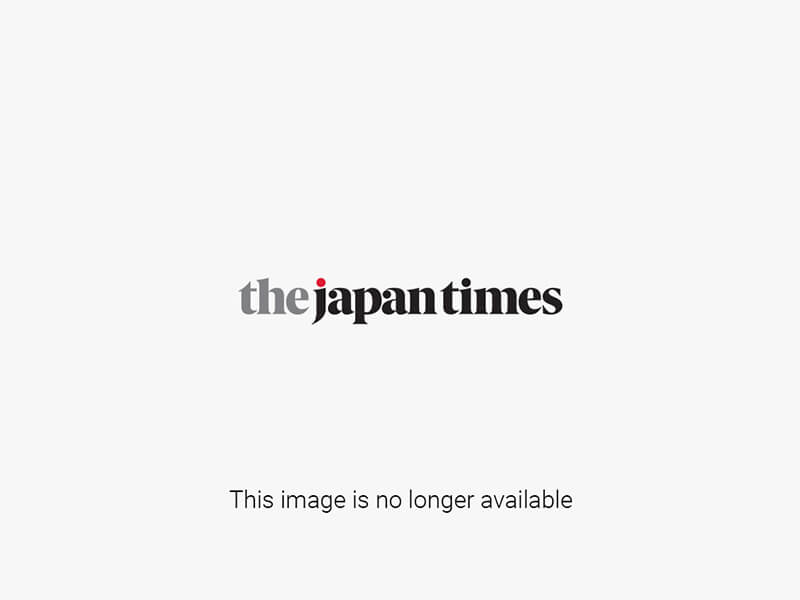The image captures a young ballet dancer, likely around 10 to 12 years old, posing after a performance on a wooden stage with floorboards running horizontally. The dancer, who has light skin and short black hair, is wearing an all-white costume consisting of white tights, white ballet shoes, and a loose, frilled shirt with elaborate cuffs. A floral vest with blue and pink flowers adorns the shirt. The dancer, who wears a hint of eyeliner accentuating their large eyelashes, smiles warmly at the audience. In a celebratory pose, they kneel on the ground with one leg bent and the other extended in a half split, one hand placed confidently on their hip and the other raised in the air. The stage background features a white tarp and partially drawn curtains, appearing purple due to the lighting, which also casts a slight reflection of the dancer on the polished wooden floor.